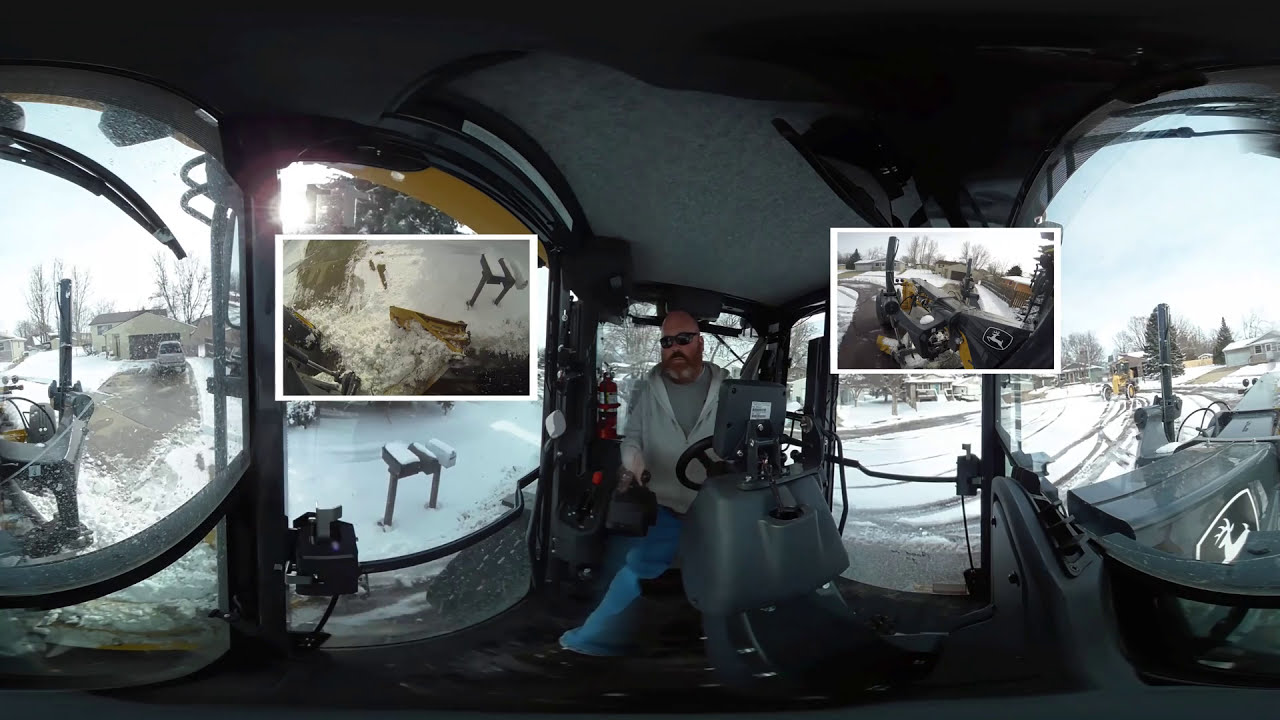In this detailed image, we see a bald man with dark sunglasses, a reddish-brown and silver mustache and beard, sitting in the center of a large, dark gray John Deere tractor's cab. He is wearing a gray hooded sweatshirt and blue jeans, which look like bell bottoms. The tractor's cabin has several large, round windows on both sides, offering a panoramic view of a snow-covered residential area with houses, mailboxes, and vehicles in driveways. The man is behind a black steering wheel, positioned in front of a gray console with a screen. A black box with a handle and a black circular knob sits to his right. Two overlaid pictures are positioned inches from his head on both sides, showing a close-up of what appears to be a snow blade and part of the tractor’s control panel. In the background, the John Deere logo featuring a white deer with antlers is visible on the back end of the tractor.